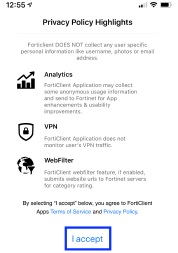This image showcases a cell phone screen displaying the privacy policy highlights for an application named "FortiClient." 

Set against a white background, the upper portion of the screen shows standard mobile icons in black: the time (12:55), a signal strength indicator resembling a bar graph, Wi-Fi, and battery status icons.

Below these, the text in black starts with "Privacy Policy Highlights." It states that the FortiClient app does not collect any user-specific personal information such as email, username, photos, or email addresses. A bar graph icon represents 'Analytics', indicating that the FortiClient application may collect some anonymous usage information and send it to Fortinet for app enhancements and improvements.

Further down, a shield with a lock icon underscores that the FortiClient application does not monitor users' VPN traffic. Additionally, a world icon with a filter suggests a 'Web Filter' feature provided by FortiClient.

The document concludes by stating, "By selecting I accept below, you agree to FortiClient's apps," followed by options to review the "Terms of Service" and "Privacy Policy" in blue text. At the bottom, there is a prominent blue button labeled "I Accept."